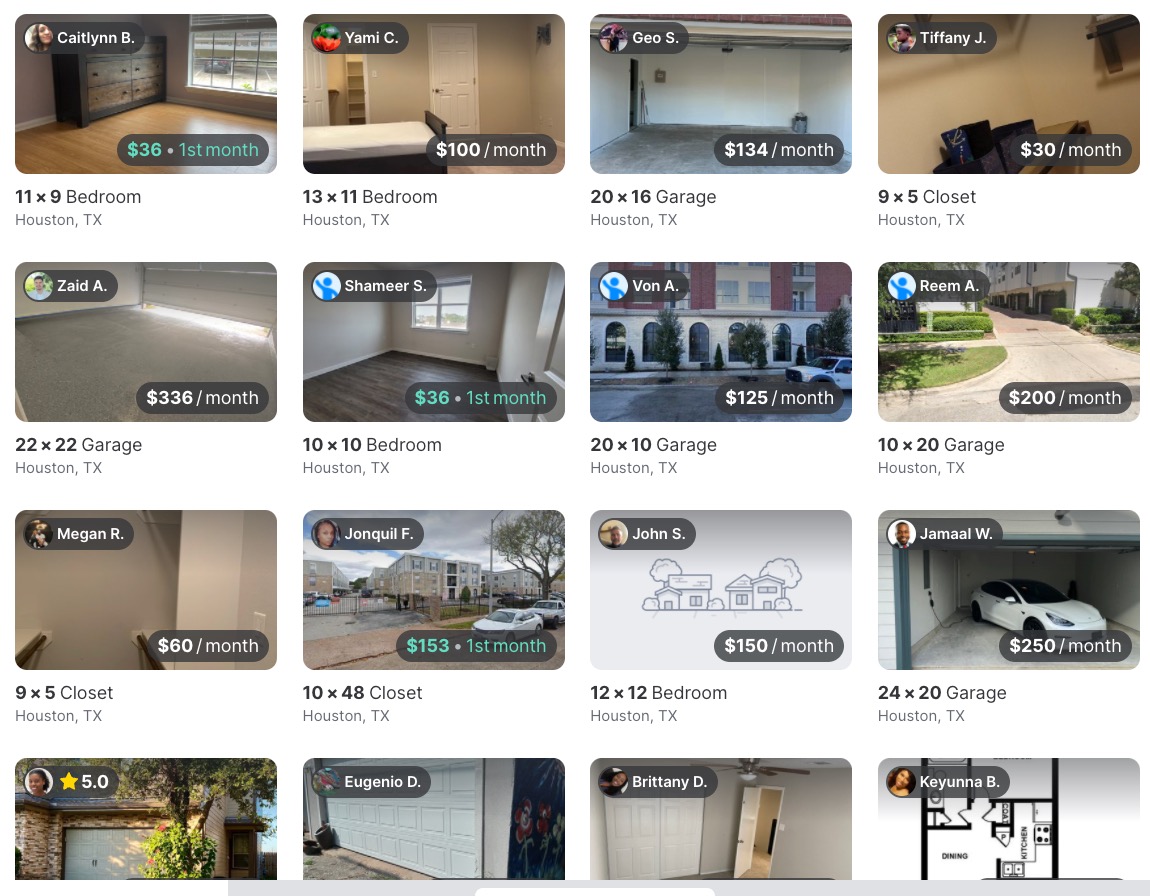The screen displays a grid of 16 thumbnails, each depicting various rental listings in Houston, Texas. The thumbnails have either an avatar or a photo of the listing's owner, along with a brief description and price for the items available. The listings include different types of spaces such as a bedroom measuring 11 x 9 feet available for $36 for the first month, a 13 x 11 feet bedroom for $100 a month, and a 20 x 16 feet garage for $134 a month. Other spaces listed include a closet for $30 a month and a larger 22 x 22 feet garage for $336 a month. Another listing features a 10 x 10 feet bedroom for $36 for the first month, and there is also a sizable 24 x 20 feet garage available for $250 a month. The listings seem to cater to various storage and rental needs, offering a range of spaces at different price points.